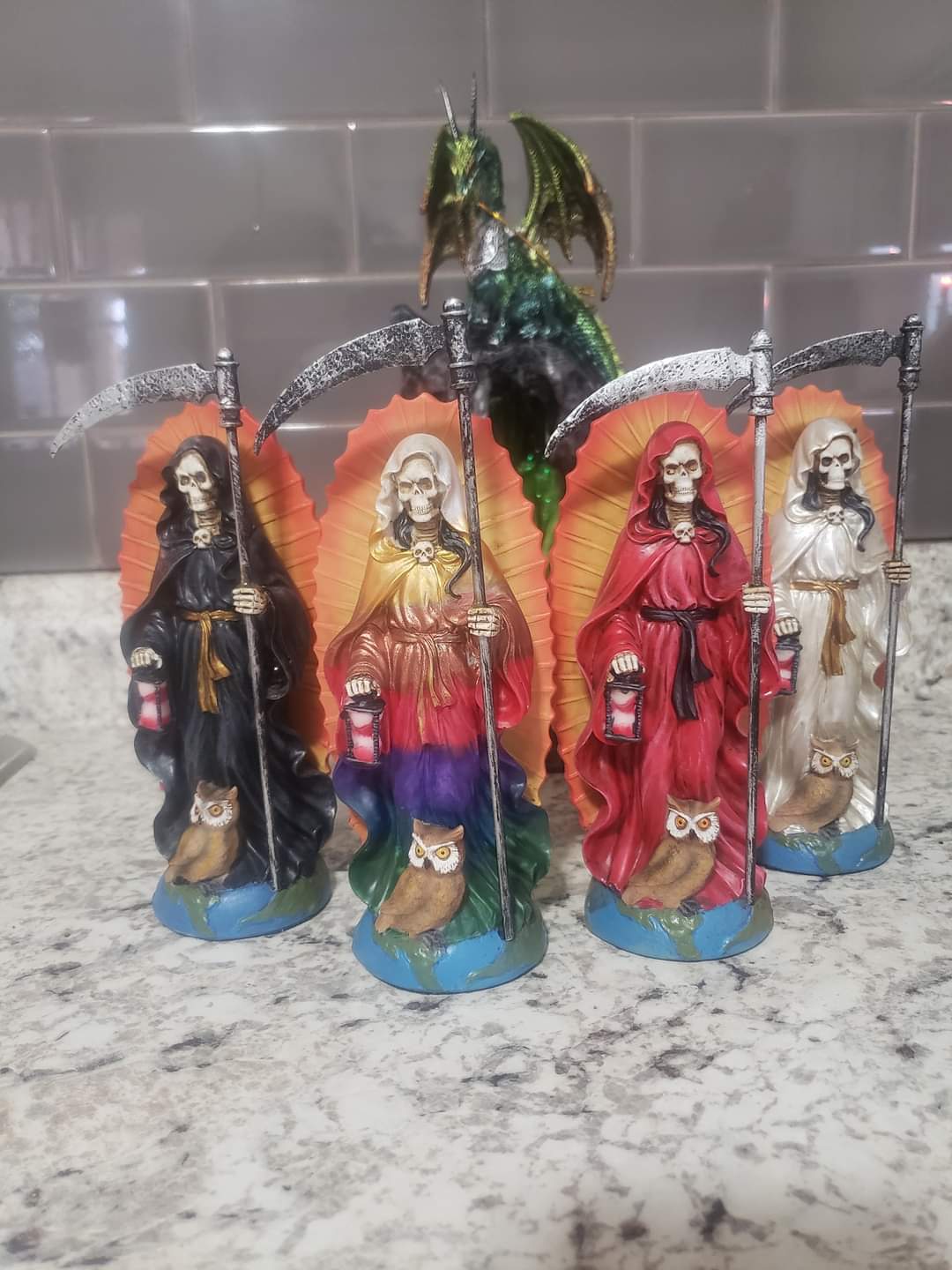The image features a collection of four intricately painted skeleton sculptures, each depicted as the Grim Reaper, standing in a row on a white marble countertop with distinctive black specks. Each skeleton holds a large scythe vertically over their head, a red lantern, and stands beside an owl on a base resembling a cut-off section of planet Earth. The first skeleton is dressed in a black robe with a gold ribbon. The second sports a vibrant multicolored robe featuring hues of yellow, red, purple, green, and blue. The third wears a red robe, has long brown hair, and a brown belt. The final skeleton at the far right is garbed in a white robe accented with gold around the belt. Behind the row of Grim Reapers, a green monster figure, possibly a dragon, with gold highlights can be seen. This setup is placed indoors against a gray tile backsplash that resembles brick.